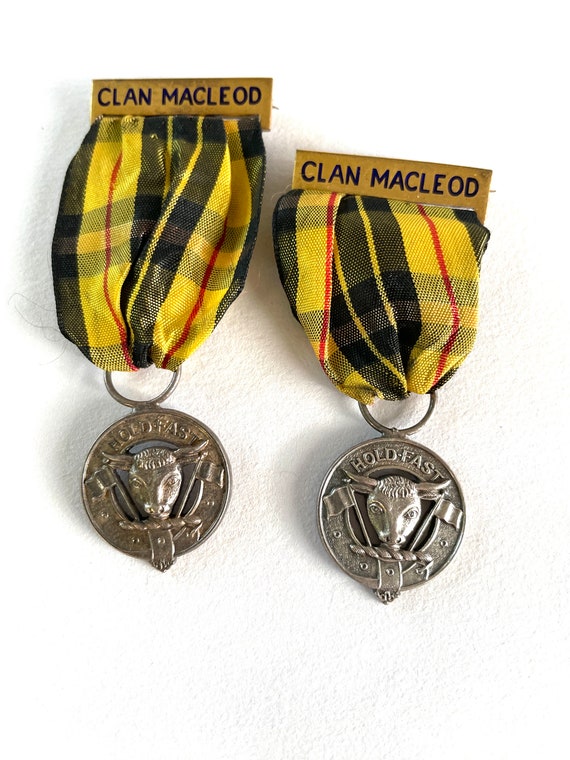The image depicts two identical silver medals positioned side by side, with the one on the left slightly higher. Each medal features a circular centerpiece displaying a bull’s head with small horns staring directly ahead. Flanking the bull are two flags, each attached to a flagpole, and the phrase "Hold Fast" is engraved along the top edge of the circular part. Below this, a piece of cloth, folded to serve as the handle, is present, adorned in a plaid pattern with primary colors of yellow and black interwoven with small red stripes. Above this fabric is a gold rectangular plate inscribed with "Clan Macleod" in black capital letters. The medals are connected by a hoop to the fabric, which appears functional as either a neck ribbon or for wall display. The silver medals, complete with their ornate design and inscribed elements, encapsulate the heritage of Clan Macleod.